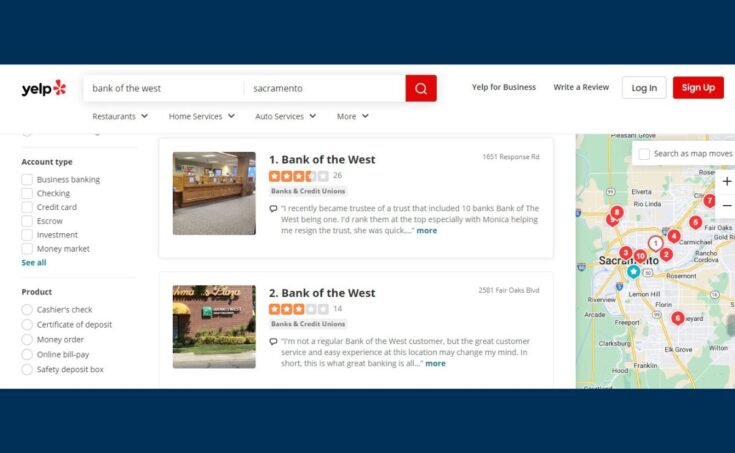The image showcases a Yelp search for banks in Sacramento, with the focus on finding a new banking option. The map on the right-hand side highlights Sacramento, pinpointing the search results. The specific bank under consideration is Bank of the West, seemingly a local Sacramento chain. Yelp lists 10 branches in the area, with the screenshot displaying the first two entries, both of which have approximately three-star ratings. The reviews suggest a common trend where banks often receive moderate ratings, typically driven by customers sharing negative experiences.